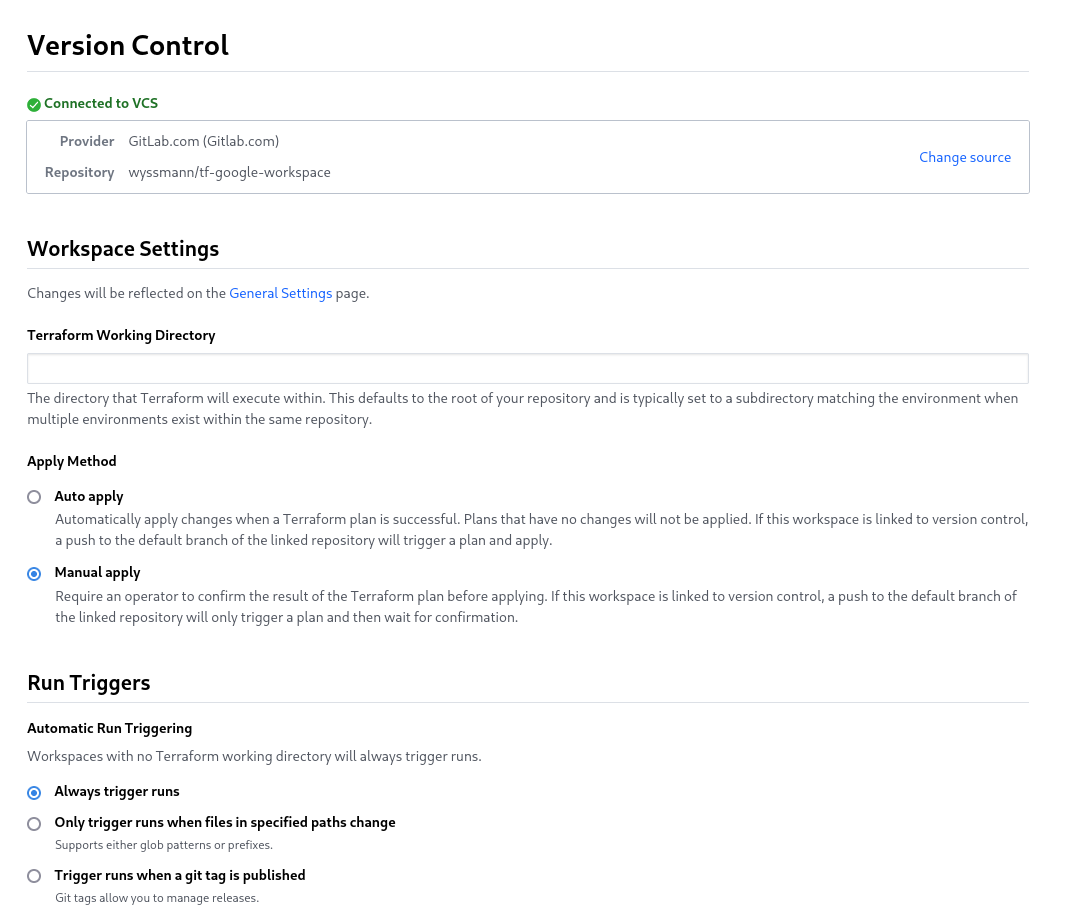This screenshot taken from a website features a clean, white background with no graphics, emphasizing the textual details prominently. At the upper left-hand corner, there is a heading "Version Control" displayed in bold black font. Directly beneath it, "Connected to VCS" is written in green font, accompanied by a green circle with a white checkmark to its left, signifying a successful connection. Below this, in grey font, the label "Provider" appears with the subsequent detail "GitLab.com." Further down, under "Repository," the web address of the repository is listed.

A secondary bold headline "Workplace Settings" is found below this, followed by another bold headline, "Terraform Working Directory." Underneath, a brief description is provided in grey font.

Continuing down, another heading in bold black font reads "Apply Method," which includes two options. The first option, "Auto Apply," is followed by a brief description in grey font. The second option, "Manual Apply," is selected, indicated by a blue-highlighted circle to its left.

At the very bottom of the screenshot, the heading "Run Triggers" is visible. Below it, there are three options available, with "Always Trigger Runs" being the selected choice. 

This structured textual interface appears to detail settings for version control and configurations for a workspace, highlighting various options and their current selections.